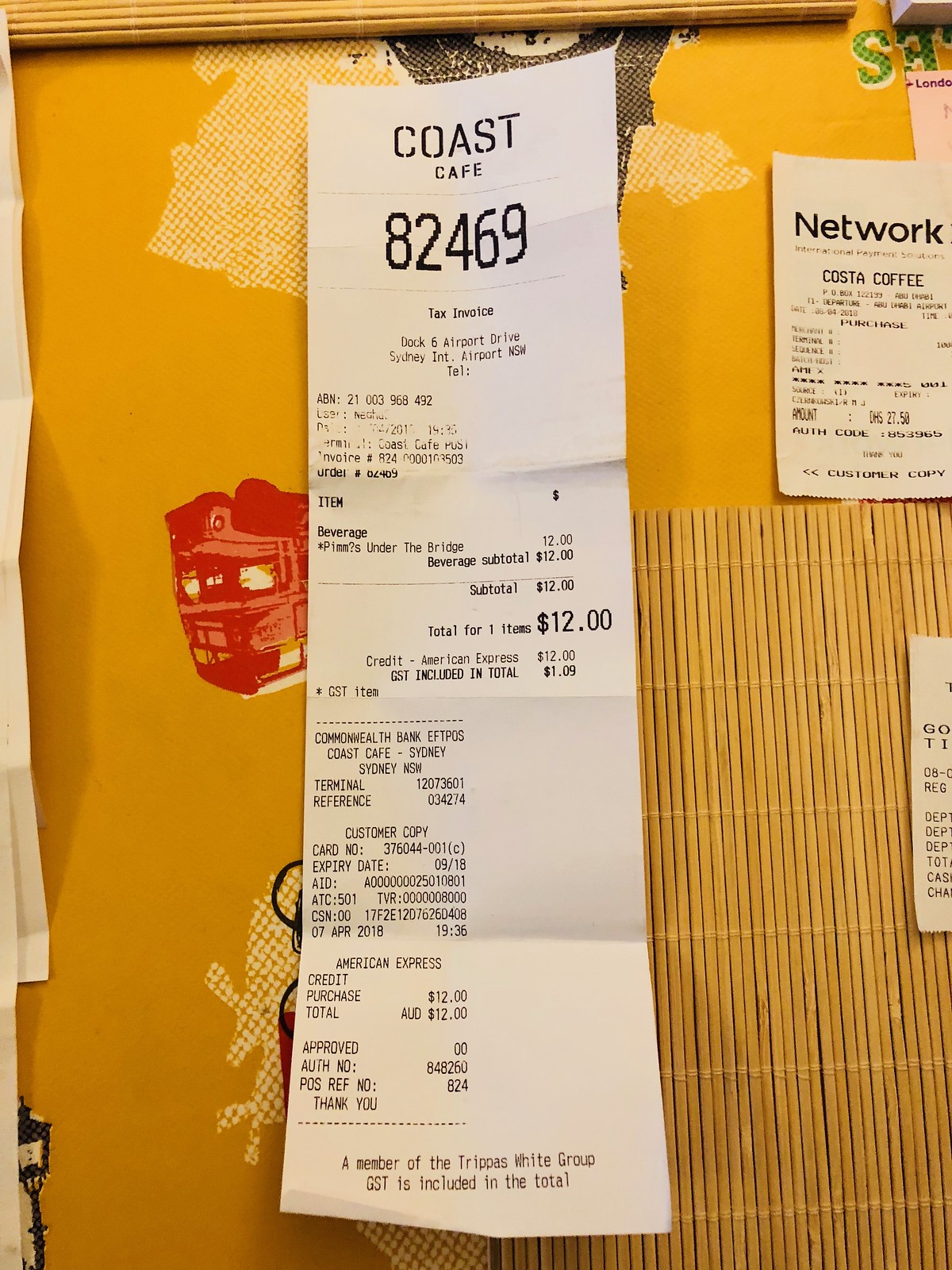This photograph features three overlapping receipts placed on a decorative placemat with colors of gold, red, yellow, and white. The focal point is a large receipt from Coast Cafe, prominently displaying a transaction number "82469" and labeled as a Tax Invoice. This receipt, originating from Dock 6, Airport Drive, Sydney International Airport, details the purchase of a $12 beverage charged to an American Express card. Additional miscellaneous writing is found below the main details. Adjacent to this receipt, slightly to the right, is a smaller receipt from Costa Coffee, noted with the term "Network," although the details are somewhat indistinct. Another receipt lies partially visible beneath these two. The placemat features modern art designs and a bamboo roll, possibly for sushi-making, extends into the upper part of the frame, adding a unique texture to the composition.